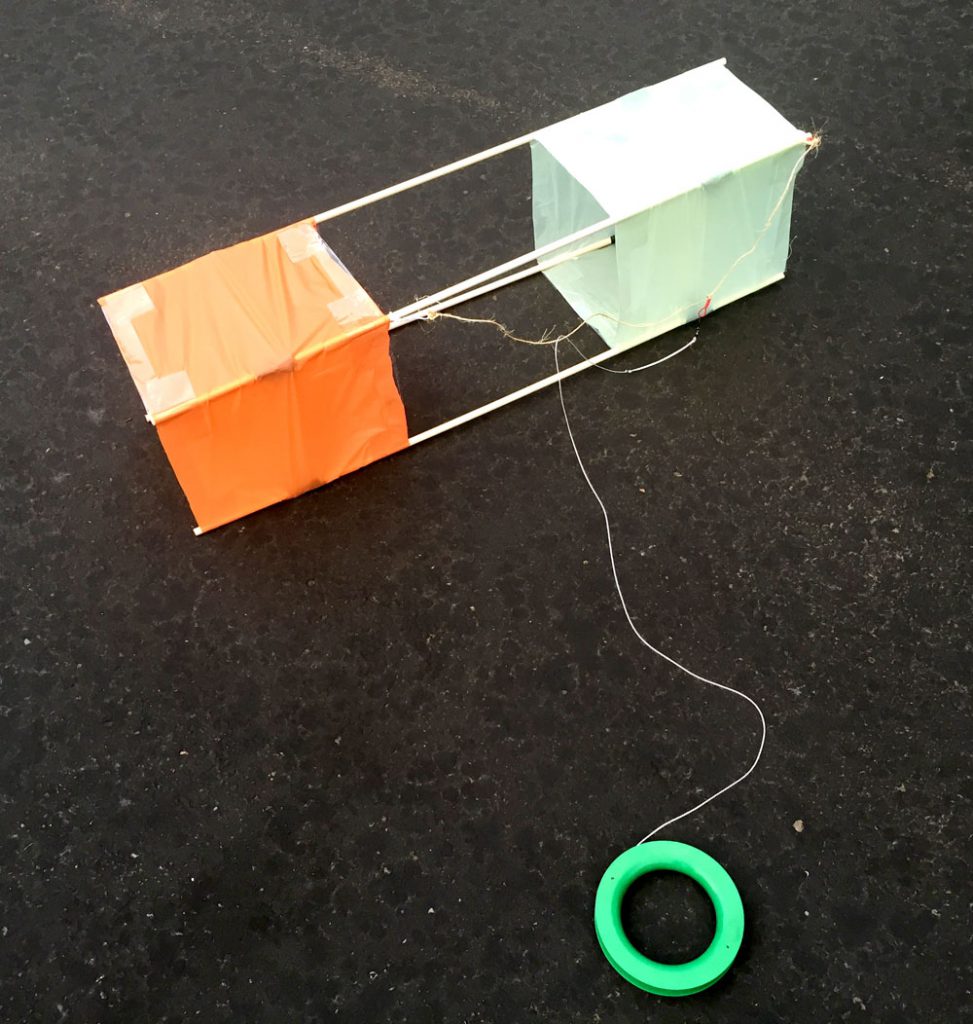This photograph captures a rectangular structure, resembling a box kite, positioned on a dark, asphalt surface. The kite features two cube-shaped sections, with the left cube being orange and the right cube being a light green. These cubes are connected by four thin wooden poles, forming an open middle section between them. A white string extends from the structure and leads down to a perfectly round, lime-green circular handle, likely used to control the kite. The ground beneath the kite shows patches of darker colors, indicating variances in the asphalt surface. The overall setup suggests that this could be a type of box kite, although it remains grounded, possibly hinting at potential issues with flight or just capturing the moment before takeoff.